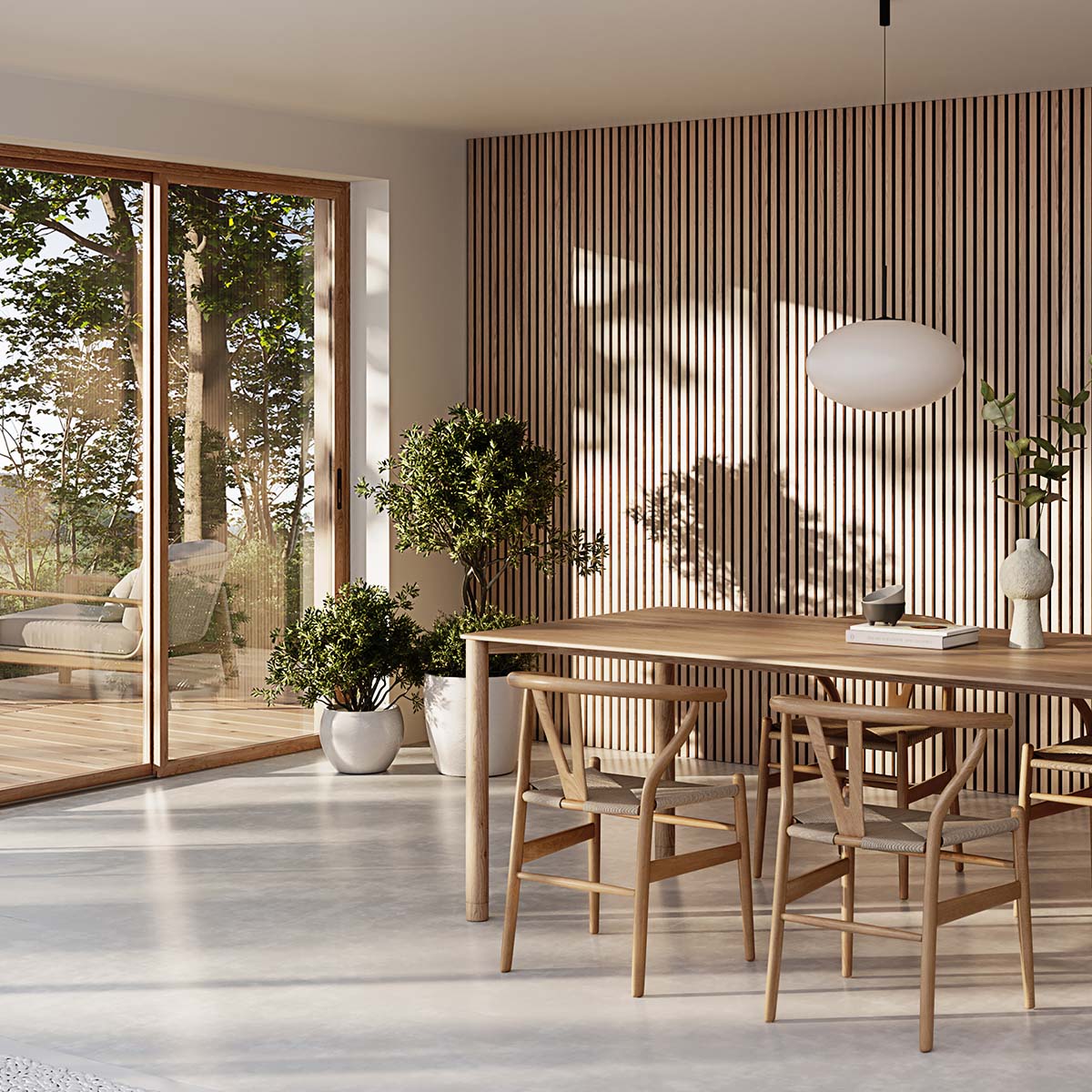The image features a clean, modern dining room with a minimalist aesthetic. The back wall is composed of vertical wooden slats, which provide a natural, textured backdrop. Light filters in through a large sliding glass door on the left, casting intricate shadows onto the slatted wall. Near this door, two potted plants add a touch of greenery; one is a taller plant with another smaller plant sharing the same pot, and the other is a more modestly sized pot set nearby.

The light-colored wooden dining table, which appears to have a thin, simple design with slim legs, is surrounded by four matching chairs. The seats of the chairs are crafted from twine or ribbon-like material, bringing an artisanal quality to the space. On the table, there's a white vase holding a sprig of flowers, a book with a white binding, and a small decorative dish.

Above the table hangs a white globe lamp suspended by a single cord, providing a soft, ambient light. The floor appears to be a single piece of light-colored polished concrete, enhancing the simplicity and elegance of the room. In the bottom left corner, a partially visible rug adds a hint of texture.

Beyond the sliding glass door is a deck, where an outdoor chair with upholstered cushions is visible, and beyond that, a view of trees adds to the serene, nature-inspired atmosphere of the space. The overall feel is one of modern simplicity combined with natural elements, creating a tranquil and inviting dining environment.